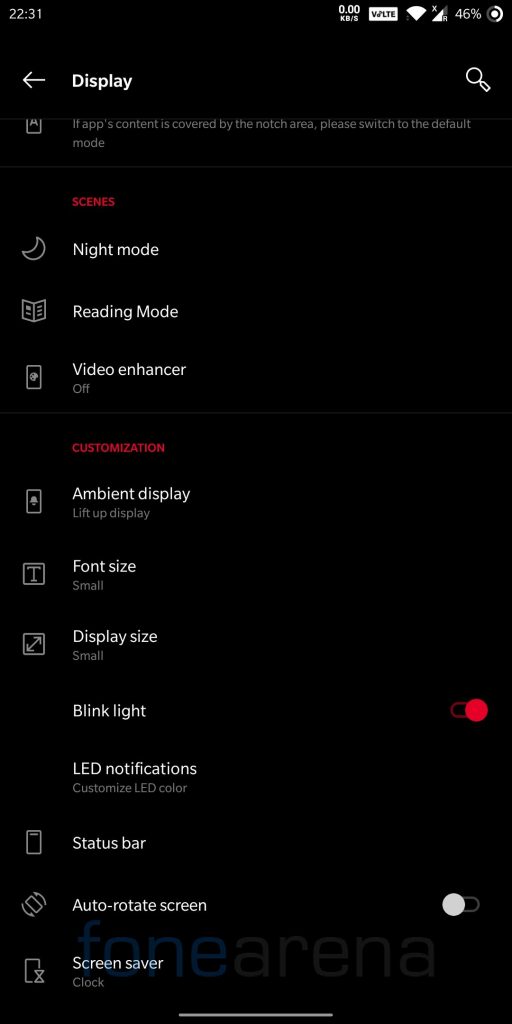The image showcases a smartphone display against a black background. The device screen prominently shows the time as 22:31 at the top, along with various status indicators on the right-hand side including signal strength, Wi-Fi signal, battery life, and other icons.

Beneath the status bar, the display settings menu is visible. The heading "Scenes" is highlighted in red, followed by icons and text for different modes: Night Mode, Reading Mode, and Video Enhancer. Below these options, another red heading labeled "Customization" appears, featuring several icons and descriptions for settings such as Ambient Display, Font Size, Display Size, Blink Light (without an icon), LED Notifications (without an icon), Status Bar, Auto-Rotate Screen, and Screen Saver.

The Blink Light setting has a red toggle switch positioned to the right, indicating that it is enabled. Conversely, the Auto-Rotate Screen setting features a white toggle switch set to the left, signifying that it is disabled.

Superimposed at the bottom of the image is the branding "PhoneArena," with "FONE" in blue and "arena" in grey.